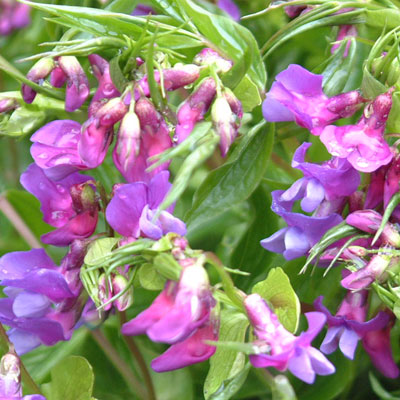This close-up photograph captures a vibrant outdoor scene, possibly from the wild or a personal garden, focused on a collection of delicate flowers surrounded by lush greenery. The central and most striking elements are the numerous flowers, which range from a soft lilac to a vivid fuchsia in color. The flowers have an upside-down, bell-shaped structure with a gradient effect, transitioning from light pink at the petal edges to a deeper purple near the base. Some flowers also reveal glimpses of white emanating from their centers. The flowers, both in full bloom and in various stages of budding, appear intermixed with green leaves, some of which seem slightly dilapidated. The entire image is filled with these botanical elements, showcasing a palette of pale green, purple, fuchsia, and white, capturing the intricate beauty of nature in a mesmerizing and detailed manner.